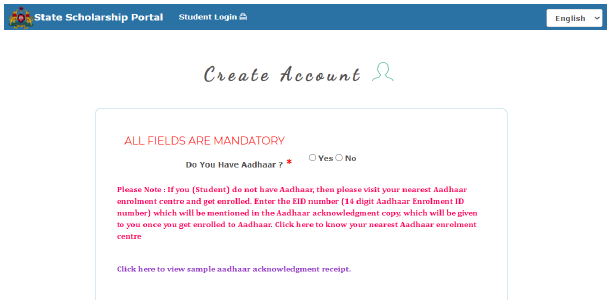**Detailed Descriptive Caption for the Image of State Scholarship Portal's Create Account Page:**

The image showcases the "Create Account" page of the State Scholarship Portal. At the top of the interface, there's a header featuring a logo placed on the top left corner. On the right side of the header, there are options for "Student Login" and a language dropdown menu that is currently set to English. Centered just below the header, the page title "Create an Account" is prominently displayed, accompanied by an icon of a person.

The main content area starts with a mandatory fields notice, indicating that all fields are required. The first field asks, "Do you have ADIHAR?" with radio buttons for "Yes" and "No" responses. An important note highlighted in red font follows, instructing students who do not have ADIHAR to visit their nearest ADIHAR enrollment center to complete their enrollment. It further explains that students should enter their EID number, a unique 14-digit ADIHAR enrollment ID found on the ADIHAR acknowledgement receipt received upon enrollment.

Additionally, the page includes a helpful link to locate the nearest ADIHAR enrollment center and another clickable link to view a sample of the ADIHAR acknowledgement receipt. Overall, the image provides a comprehensive view of all necessary steps and information required for creating an account on the portal.